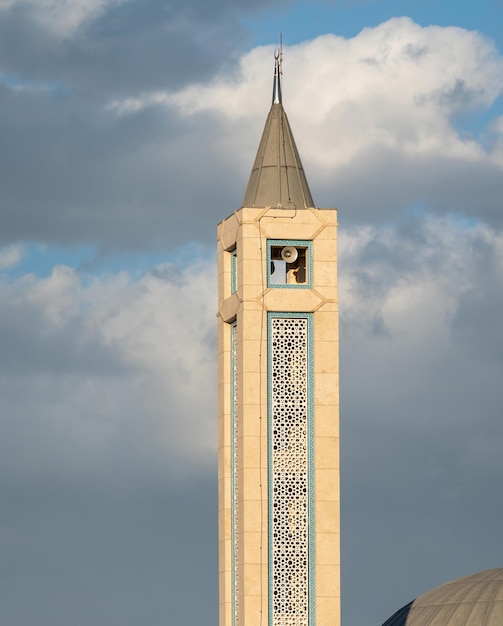The image depicts a tall tower, predominantly occupying the height of the picture, framed against a backdrop of an overcast sky interspersed with both dark and light clouds, with glimpses of blue sky peeking through. The tower, constructed of white stone or brick, stands almost like a rectangular column. It features a distinct white lattice or grill design bordered by a teal blue edge running vertically along its sides. Toward the top, an opening reveals a large speaker and a small figure standing beneath it. The apex of the tower culminates in a grey conical roof, likened to an inverted funnel, with a silver antenna protruding from its tip. The structure resembles a minaret, possibly serving a call for prayer, and hints of another building's curved roof are visible at the very lower right corner of the image, suggesting the tower is part of a larger complex. The overall ambiance is one of a cloudy, gray day, with the tower standing tall and resolute amidst the impending storm.